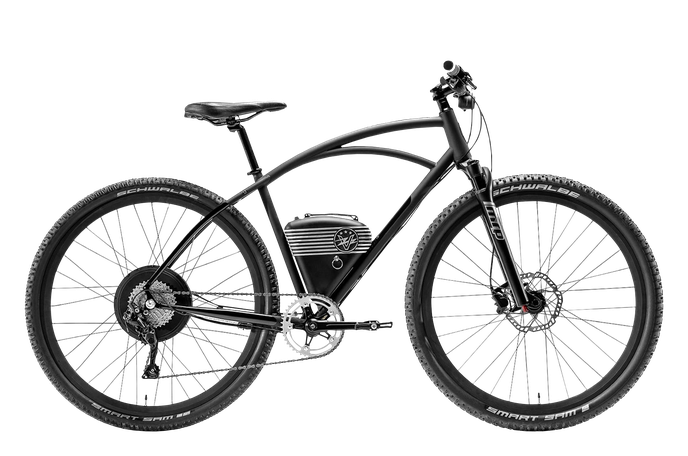This is a detailed drawing of a black electric bicycle facing to the left, set against a white background. The bicycle features a black looping frame with a steep slope and two identically sized black tires, each adorned with the name brand "SCHWALBE" in white lettering on opposite sides. Both wheels are equipped with silver spokes. The bike has black female handlebars with brakes positioned on them and silver detailing. 

In the central section of the bicycle's frame, which creates a near-triangular shape, there is a black, triangular-shaped object with rounded upper edges. This appears to be the casing of an engine, suggesting that the bike is electric. The casing includes white horizontal stripes near the top and a round logo in the middle.

Additional features include a slightly elongated seat, typically designed for female riders, and a silver chain. There is also a basket-like structure attached to the lower bar of the frame and a chest on the side, likely intended to hold water. Lettering "M-I-P" is visible on the front part of the bike.